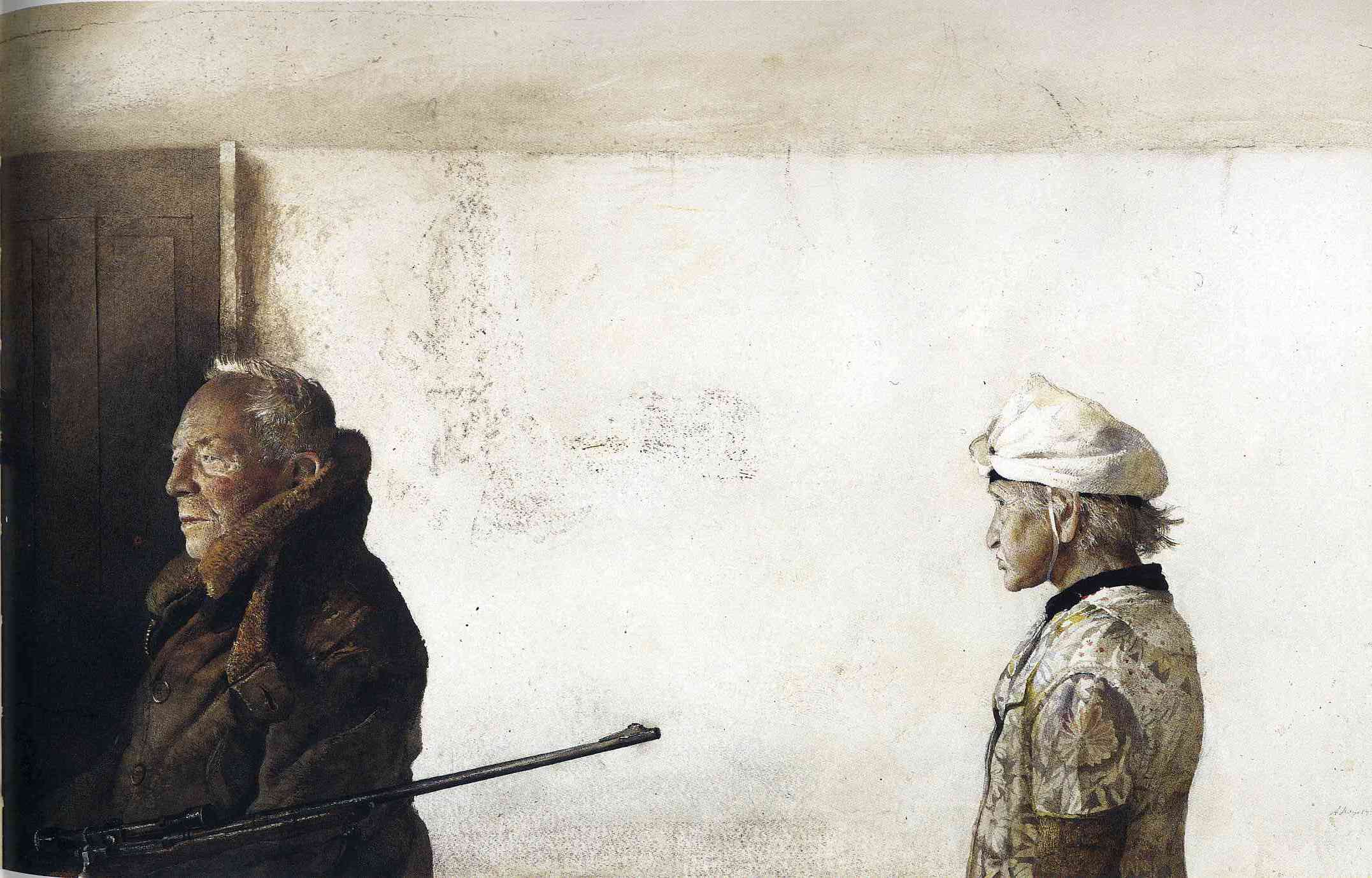This painting portrays a poignant scene between two elderly men set in a stark, barren room with a white wall and a possible door or wood paneling on the left. The man on the left is depicted in profile, deeply contemplative or focused, wearing a large, dark winter coat and carrying what appears to be a gun. His face is marked by lines and a stoic expression, indicative of determination. His hair is graying but not completely white. Standing a few strides behind him, another older man in a light short-sleeved shirt and a turban or light hat with a string under his chin gazes at the first man. His hair is also graying but is shabbier and longer. The bond or tension between these two figures, emphasized by their contrasting attire and positioning, adds a layer of depth to the emotional narrative of this artwork.